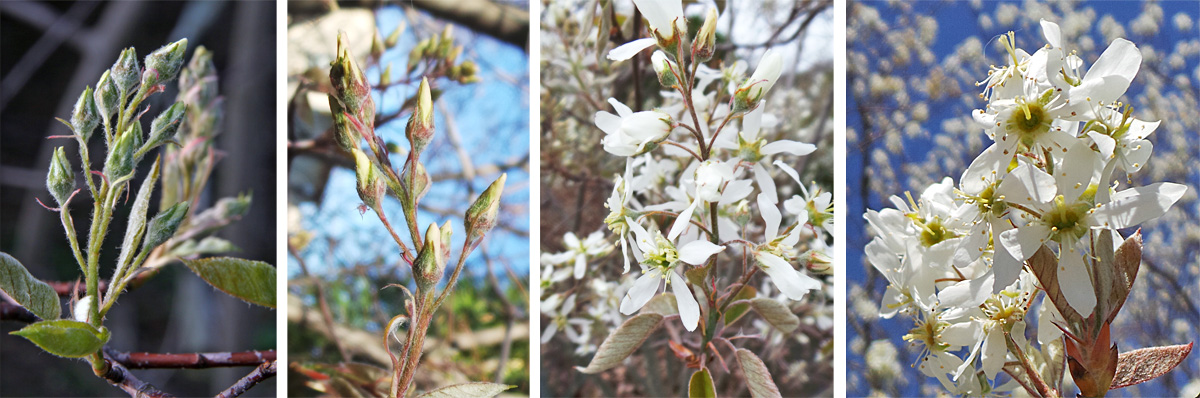This image consists of four side-by-side photographs showcasing the progressive blooming stages of a single type of flower, from left to right. In the first picture, we see green buds against a gray backdrop, representing the initial stage where the buds are just starting to appear, possibly in early spring. The second picture shows the buds beginning to lighten with hints of red details, with a light blue sky in the background. The third image captures the moment the flowers start to open, revealing white petals inside, and the background here transitions to a mix of brown and white. Finally, the fourth picture depicts the flowers in full bloom, their white petals fully opened and accented with yellow centers, set against a clear blue sky. This series beautifully illustrates the natural progression of the flower's life cycle from budding to full bloom.